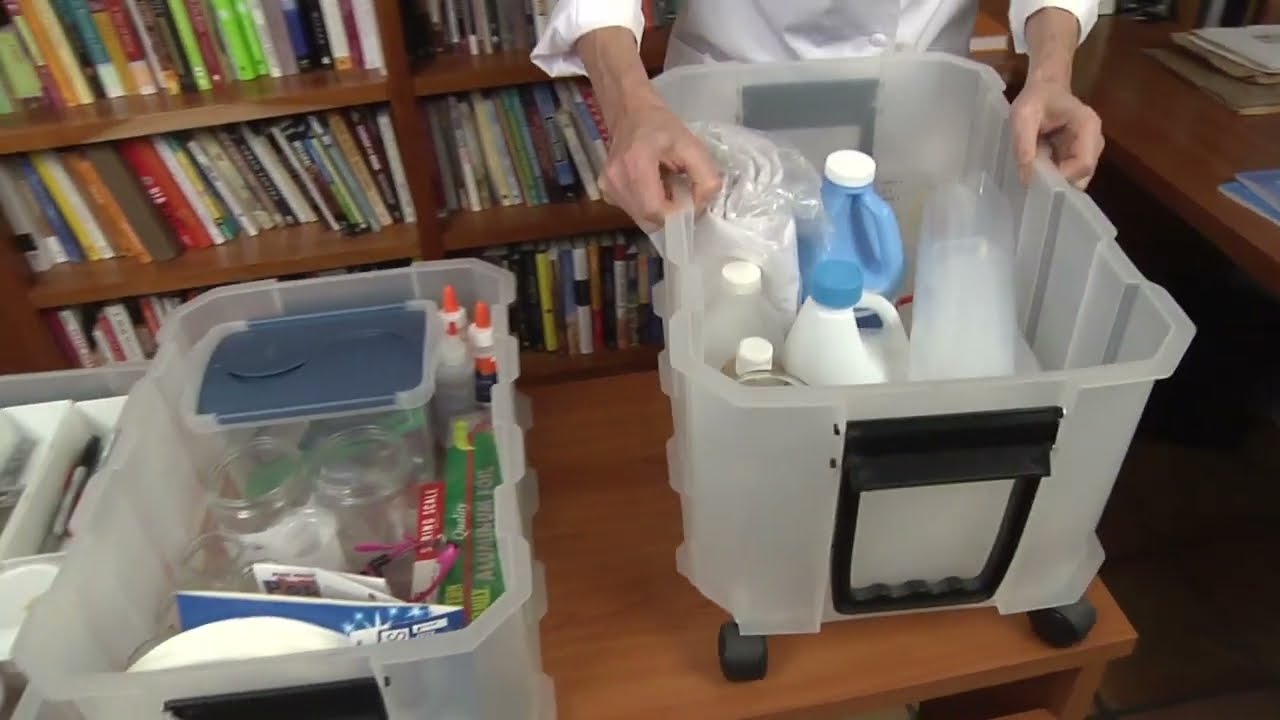In this indoor scene, a person is standing behind a wooden table, holding a large, clear white Tupperware bin with black handles. The person, dressed in a long-sleeved white shirt with rolled-up sleeves, has both hands gripping the bin, which is positioned on the table in front of them. The Tupperware bin contains various containers, including a light blue bottle with a white cap and a white bottle with a light blue cap, along with other small clear bottles. To the left of this large bin, there are two smaller plastic bins; the medium-sized bin contains items like glue, smaller containers, and papers, while the smallest bin holds containers with white tops, measuring spoons, and other miscellaneous items. Behind the table, rows of books in different colors line the shelves of a bookshelf, and on the upper right corner of the table, there is an additional smaller table with a picture on it.